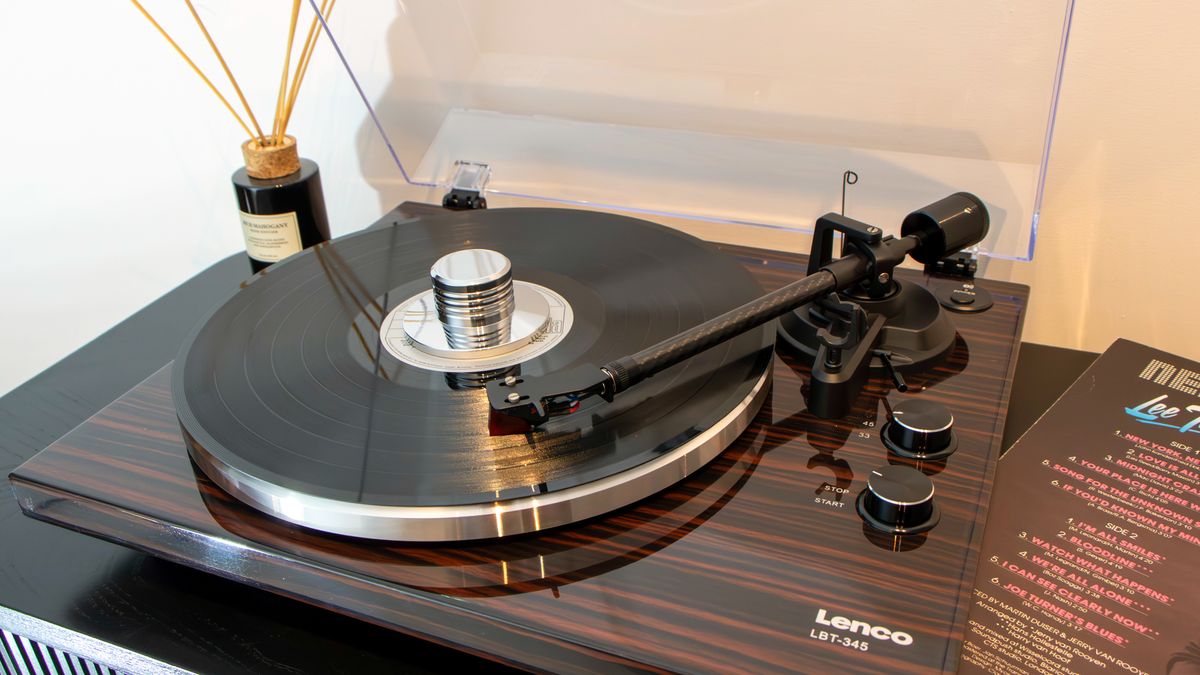This image captures a detailed photograph of an old-style vinyl record player, labeled with the brand name "Lenco" and the model number "LBT-345" in white text at the bottom right corner. The record player, characterized by its smooth, well-maintained chromed circular part and red and black striped surface, is situated in a brightly lit room with a whitewashed wall. The player’s black arm with the needle rests on the vinyl record, which is actively playing. Above the model label, two black knobs are visible, one labeled "Stop/Start" and the other displaying speed options "33" and "45". To the top left of the record player, there is a black bottle holding incense sticks. On the right side of the image, the back of the album cover is visible, listing out song titles, including "Joe Turner's Blues." The casing of the player features a black and brown pattern, and the background wall shows a light-blue hue blending into a pinkish tone towards the right.